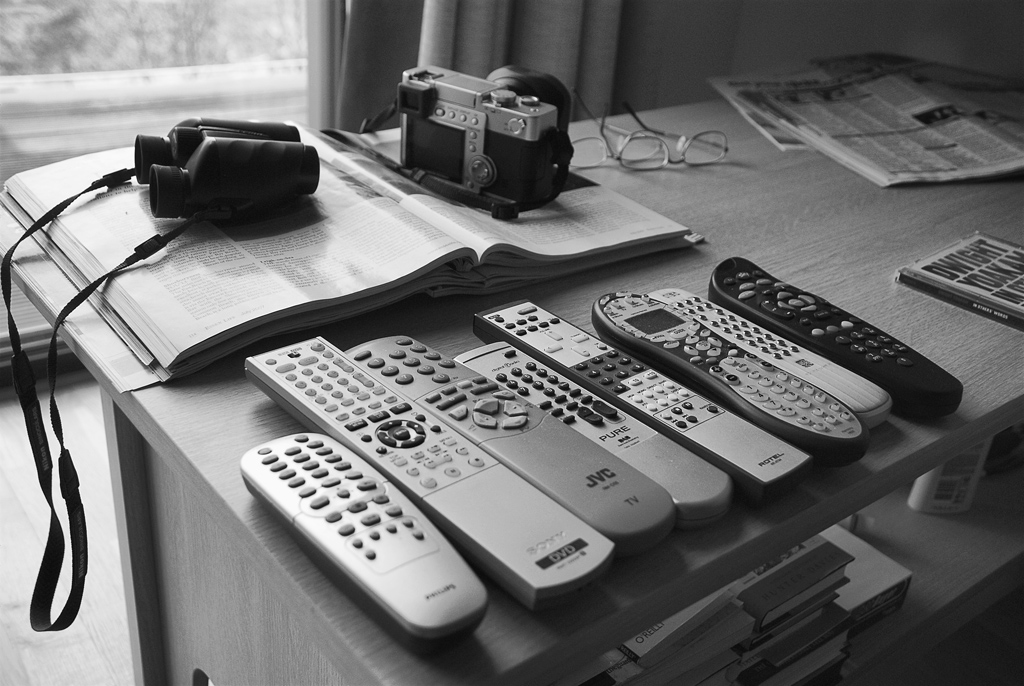This evocative black-and-white photograph captures an intricately arranged desk in what appears to be an office. Dominating the composition, a large window that extends to the ground is located in the upper left-hand corner, providing a glimpse of trees outside. The desk itself is topped with an assortment of items meticulously described by various observers. In the upper left section of the desk, an open book lies next to a pair of black binoculars, the strap of which cascades over the desk's edge. Adjacent to the book, an old-fashioned camera, resembling a Pentax K-series, sits prominently. To the right of the camera, there are one or possibly two pairs of glasses, and beside them rests a newspaper. In the foreground, eight remote controls are precisely lined up in a horizontal row, featuring brands such as Philips, Sony, and JVC, differing in lengths and colors. Notably, a CD or book bearing Dwight Yoakam's name is also visible on the desk. Below the desktop, a second shelf houses a haphazard collection of stacked paperback books and a bottle that could be glue or lotion. The photograph captures a snapshot of a cluttered yet methodically arranged workspace, infused with a sense of lived-in detail and personal touches.